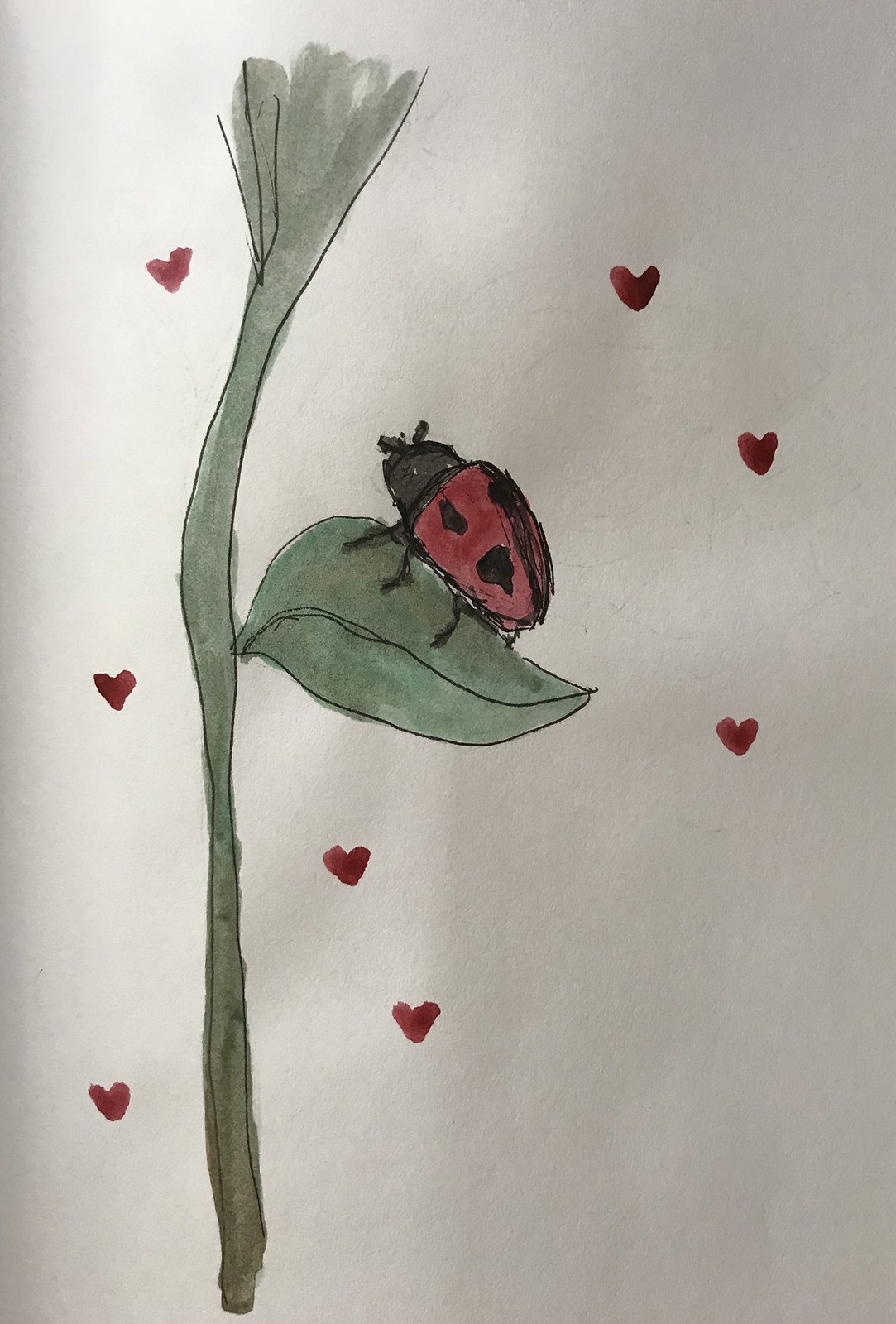In the image, a ladybug with a black head and vibrant red wings adorned with two black spots is perched gracefully on a leaf extending rightward from a tall stalk. The artwork appears to be a mixed-media piece, initially sketched with a fine-point marker or pen, and then filled in with either watercolors or marker—though the subtle variations in the green stem suggest watercolors. The background is festooned with small, red hearts that add a whimsical charm to the scene, all set against a slightly wrinkled, white piece of paper. The detailed observation of this ladybug on the leaf showcases both the artist's delicate linework and the soft, layered color application.